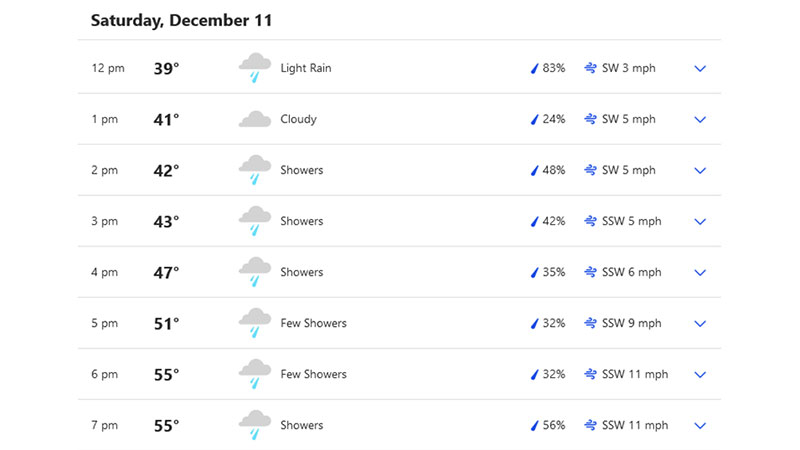The image is a screenshot taken from a weather application on a mobile device, showcasing the hourly weather forecast for Saturday, December 11. The top of the image indicates the date in bold, black text. The hourly forecast is broken down from 12 p.m. to 7 p.m., listed vertically in the leftmost column. 

To the right of each hour, the forecasted temperature is displayed in darker black text; for instance, 39 degrees Fahrenheit is noted for 12 p.m. Below the temperature column, small weather icons depict the expected conditions: primarily light rain or showers, with the exception of 1 p.m., which merely shows cloudy skies without any rain. 

There is a light gray line separating each hour's forecast, delineating the sections clearly. The next column provides the probability of precipitation, with 83% marked for 12 p.m., gradually varying through the day. This is followed by information on wind strength and direction, where, for example, the 12 p.m. slot lists a southwest wind at 3 miles per hour.

Finally, the last column includes downward-pointing arrows for each hour, though their specific purpose isn't described. Each row for subsequent hours adjusts the numbers accordingly for temperature, precipitation, and wind details, presenting a comprehensive view of the day's weather.